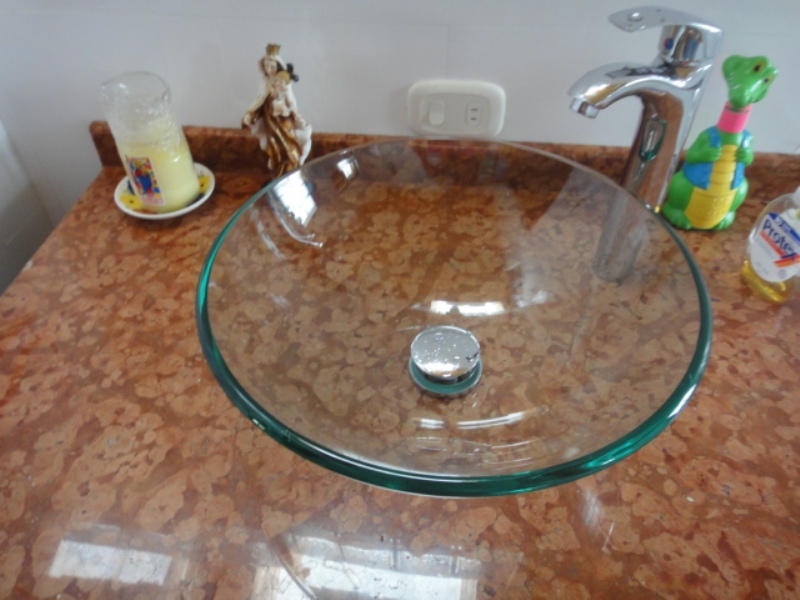The image depicts a uniquely designed sink setup that captures attention through various distinctive features. The sink itself consists of a clear glass bowl basin, uniquely positioned above the countertop instead of being recessed. This transparent bowl adds a modern touch to the ensemble. To the right of the basin, a single silver metal spigot with a minimalist design allows for temperature and spray size adjustments by shifting the handle left or right.

Behind the basin is a somewhat ambiguous white panel that might contain a small switch or an international plug, adding a curious element of intrigue. The vanity counter beneath the glass bowl showcases an unusual rusty brown splatter pattern, which, though unconventional, contributes to the overall uniqueness of the setting.

On the countertop, several intriguing items are arranged. A white candle with a lid sits on a little saucer, accompanied by a quirky ceramic pirate figure. To the right, a bottle of Protex soap and a possibly kid-friendly soap dispenser shaped like a green alligator wearing a red neck brace and a blue open vest add whimsical charm to the decor. The sink area also reflects the ambient light, possibly from one or two nearby windows, enhancing the visual complexity of the scene.

Overall, this sink setup deviates from the norm, offering both a modern aesthetic and an eclectic mix of decorative elements.